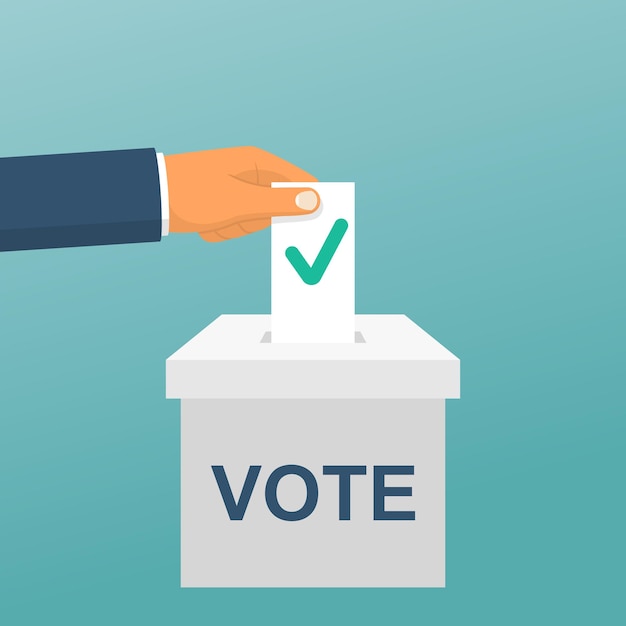This image, designed in a cartoon style, serves as an advertisement encouraging people to vote. Set against a light blue background, a central element is a white box prominently labeled "VOTE" in bold blue capital letters. The box features a slit on its top, through which a white piece of paper with a large green checkmark is being inserted. This paper is held by a hand extending from the left side of the image. The hand is clad in a blue sleeve with a white shirt peeking out from beneath, suggesting a formal attire. The overall simplicity and clarity of the image focus solely on the action of voting, with no additional text or distractions.